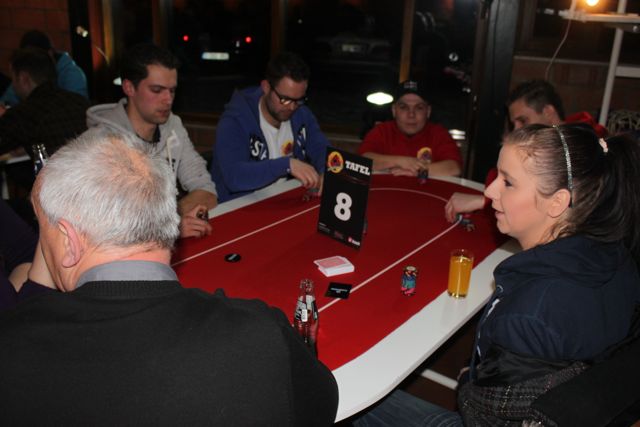This photograph captures a scene at a dimly-lit poker table, designated as table number eight, where five men and one woman are gathered, preparing to start a card game. The oval-shaped table features a distinctive red surface with a white border and a white stripe running through the middle. At the center of the table sits a deck of red and white cards, surrounded by poker chips and drinks belonging to the players. The woman, positioned on the right side of the image, has brown hair tied in a ponytail and is dressed in a black hoodie. In front of her, there is a glass of amber-colored liquid, likely beer. The man visible at the bottom left shows only the back of his head and shoulders; he is wearing a black sweater over a gray shirt and has white hair. In the background, another table and various items can be faintly seen, contributing to the overall dark ambiance of the photograph.